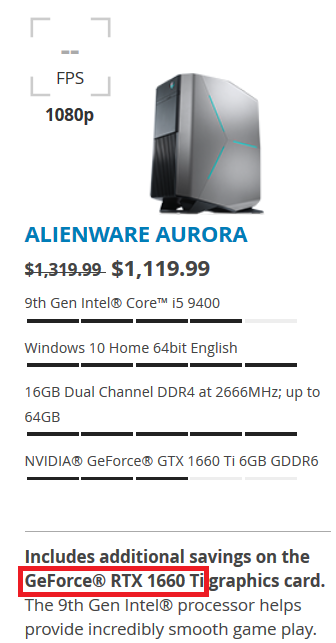The image depicts a detailed advertisement for an Alienware Aurora computer system. The portrait-oriented photo is set against a clean, white background with no defined borders on the outside. In the top left corner, there is a minimalist frame outline comprised of right-angle corners, within which "FPS" is written in black font, followed by "1080p" in smaller black text below. 

To the right of this is a sleek, gray computer tower with blue accent lines and a black frame. A prominent blue button can be seen on the tower. Below this, "Alienware Aurora" is prominently displayed in bold, blue-highlighted capital letters. 

The original price of $1,319.99 is shown crossed out, with a new price of $1,119.99 indicated beneath. The specifications listed include:
- 9th Gen Intel Core i5-9400
- Windows 10 Home Edition 64-bit (English)
- 16GB Dual Channel DDR4 at 2666MHz, expandable up to 64GB
- NVIDIA GeForce GTX graphics

At the bottom of the image, there is a promotion for additional savings on the GeForce RTX 1660 Ti Graphics card, with the "GeForce RTX 1660 Ti" highlighted in a red rectangular box. 

The overall presentation is visually organized with a clear hierarchy of information, designed to attract potential buyers with both technical details and promotional offers.